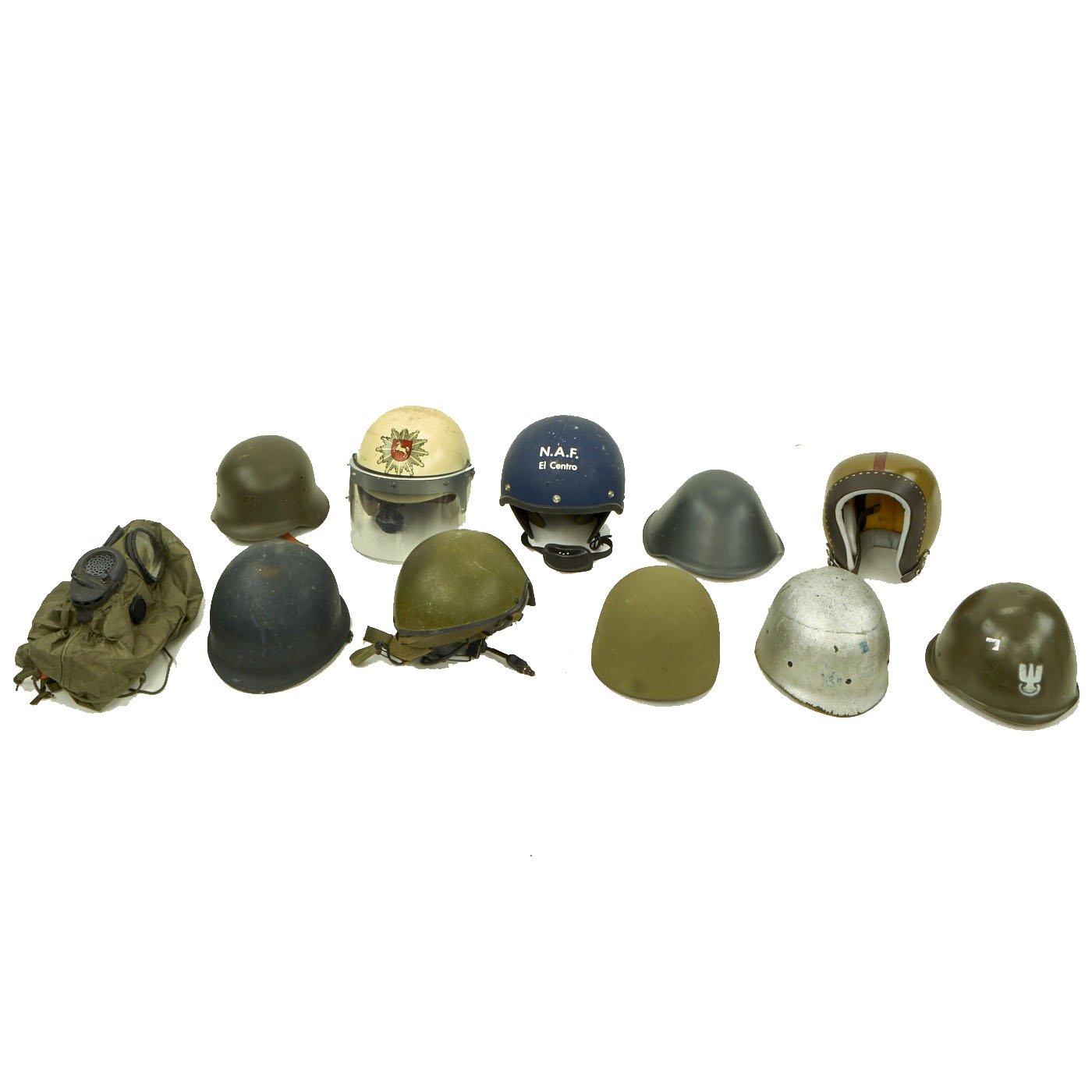The image showcases an array of eleven helmets and masks, neatly arranged in two rows against a white background. The back row, from left to right, features five helmets: a dark green helmet, a cream-colored helmet with a clear visor and a gold emblem featuring a red shield, a navy helmet marked with "N.A.F. El Centro," a gray helmet, and an old-style gray football helmet with a distinctive horseshoe opening. 

The front row starts with a green army bag positioned on the far left, followed by a black helmet, an army green helmet with a strap, another similar green helmet, a silver helmet, and concludes with an army green helmet bearing a white emblem on its front. Additionally, there’s a distinct dark green gas mask on the far left with prominent darker outlines around the eyes and mouth, alongside a string hanging from its bottom.